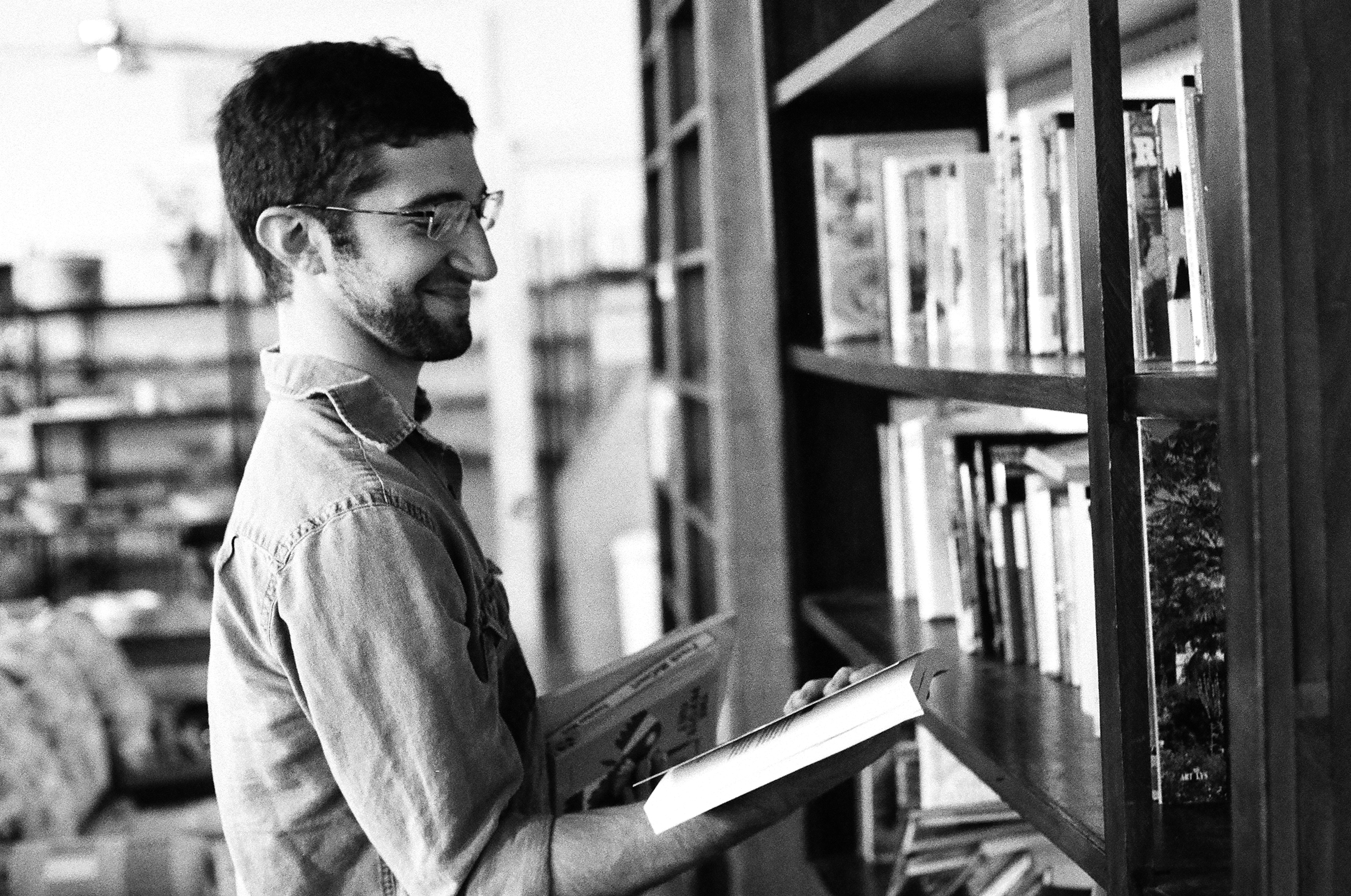In this black and white photograph, a young man stands in front of a wooden bookshelf filled with an abundant and diverse collection of books. The right side of the image is entirely occupied by the bookshelf, while the left side features the man along with more bookshelves fading into the background. Additional details like a sofa and a faint outline of a light fixture can be seen in the background, suggesting a cozy library setting. The man, who has short black hair and a hint of facial hair, is dressed in a denim button-up long sleeve shirt with the sleeves rolled up to his elbows. He is wearing black metal-framed square glasses and is engrossed in reading the back of a paperback book held in his right hand. In his left hand, he clutches a hardcover book. His expression is one of quiet enjoyment, enhanced by a slight smile as he peruses the text.